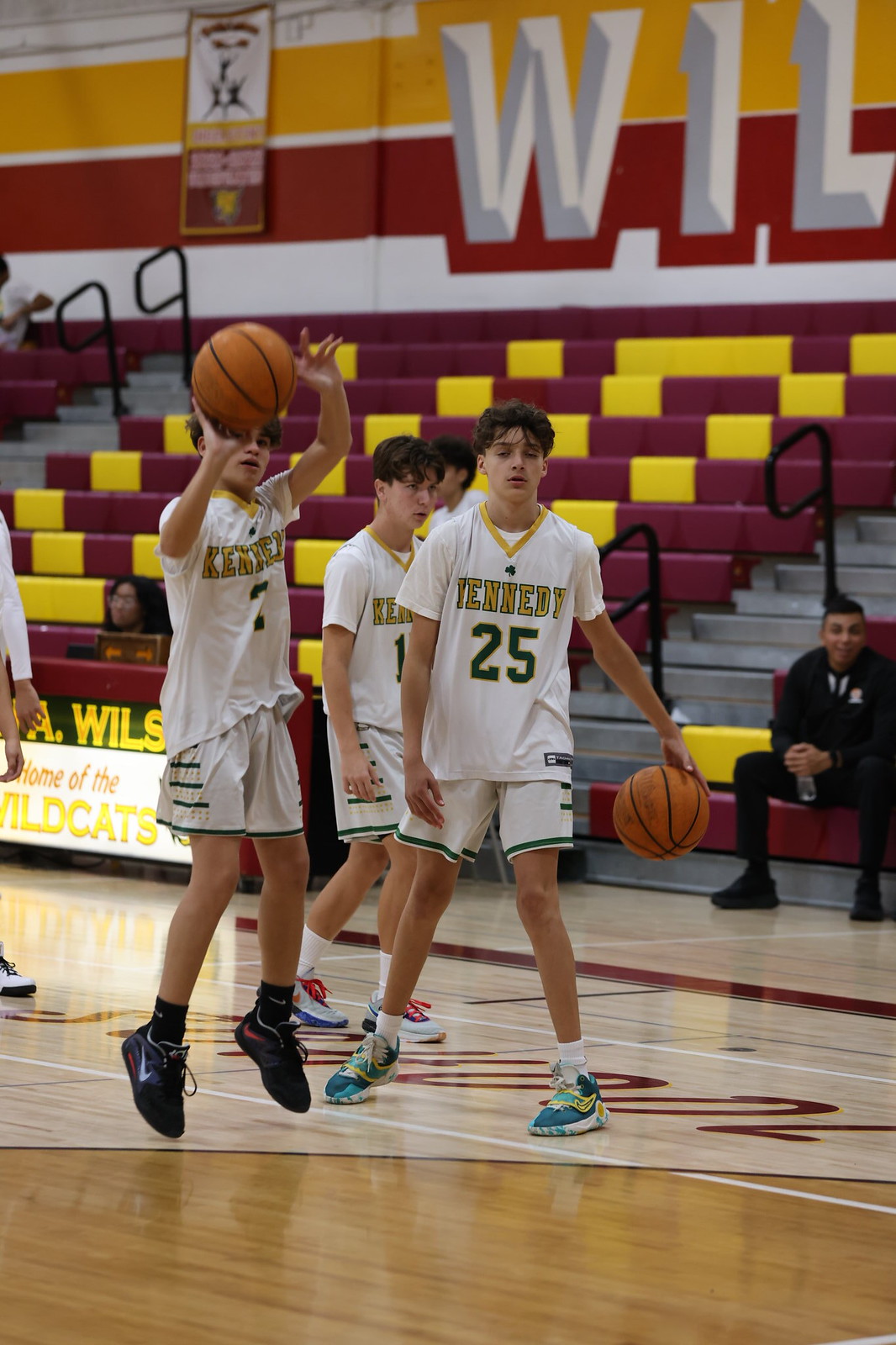This color photograph captures a close-up of a junior high basketball practice session on an indoor court. Four boys, aged approximately 13 to 14, are engaged in practice, wearing white uniforms with yellow lettering and green numbers, featuring the name "Kennedy." Each boy’s uniform also includes a yellow border around their collars and white shorts with green trims. One of the players, donning a jersey number 25 and aquamarine sneakers, is dribbling a basketball. To his left, another player, wearing jersey number 7, black sneakers, and black socks, is mid-shot, practicing from the three-point line.

The backdrop reveals the school’s burgundy and yellow bleachers, mostly empty save for a few spectators, including someone at a scorer's table with a banner reading "Home of the Wildcats," hinting at the school's mascot. The atmosphere suggests they are preparing for an upcoming game, with the scene evoking the meticulousness of a pre-game warm-up.